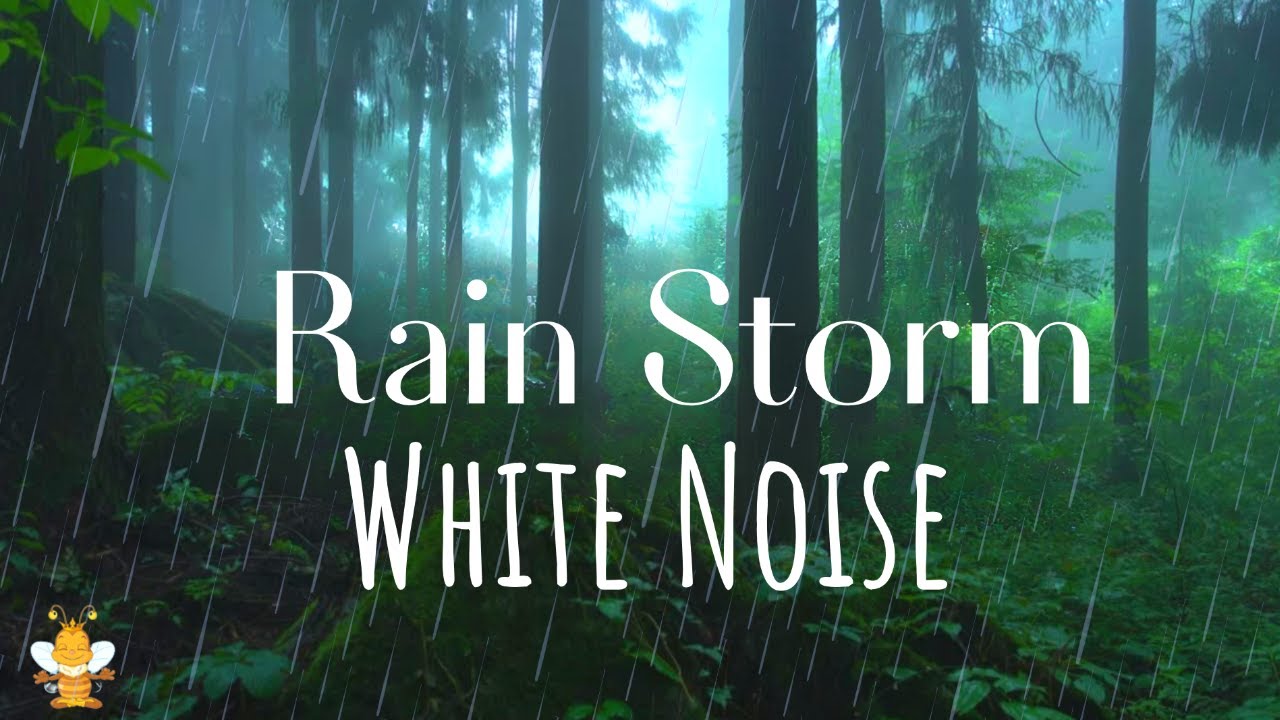This image, ideal for a YouTube video thumbnail or blog post, features a serene, illustrated forest scene teeming with green foliage and tall, brown-trunked trees. A turquoise light source emanates from the center, illuminating the backdrop of an artificial rainstorm with long, diagonal gray raindrops. Overlaying this tranquil scene is bold, white text that reads "Rainstorm White Noise" across two lines. Adding a touch of whimsy, the lower left corner showcases a cute cartoon bumblebee meditating, complete with yellow and black stripes, white wings, and expressive facial features. The entire composition creates a soothing and inviting visual designed to attract viewers seeking relaxation and calm through the sounds of nature.